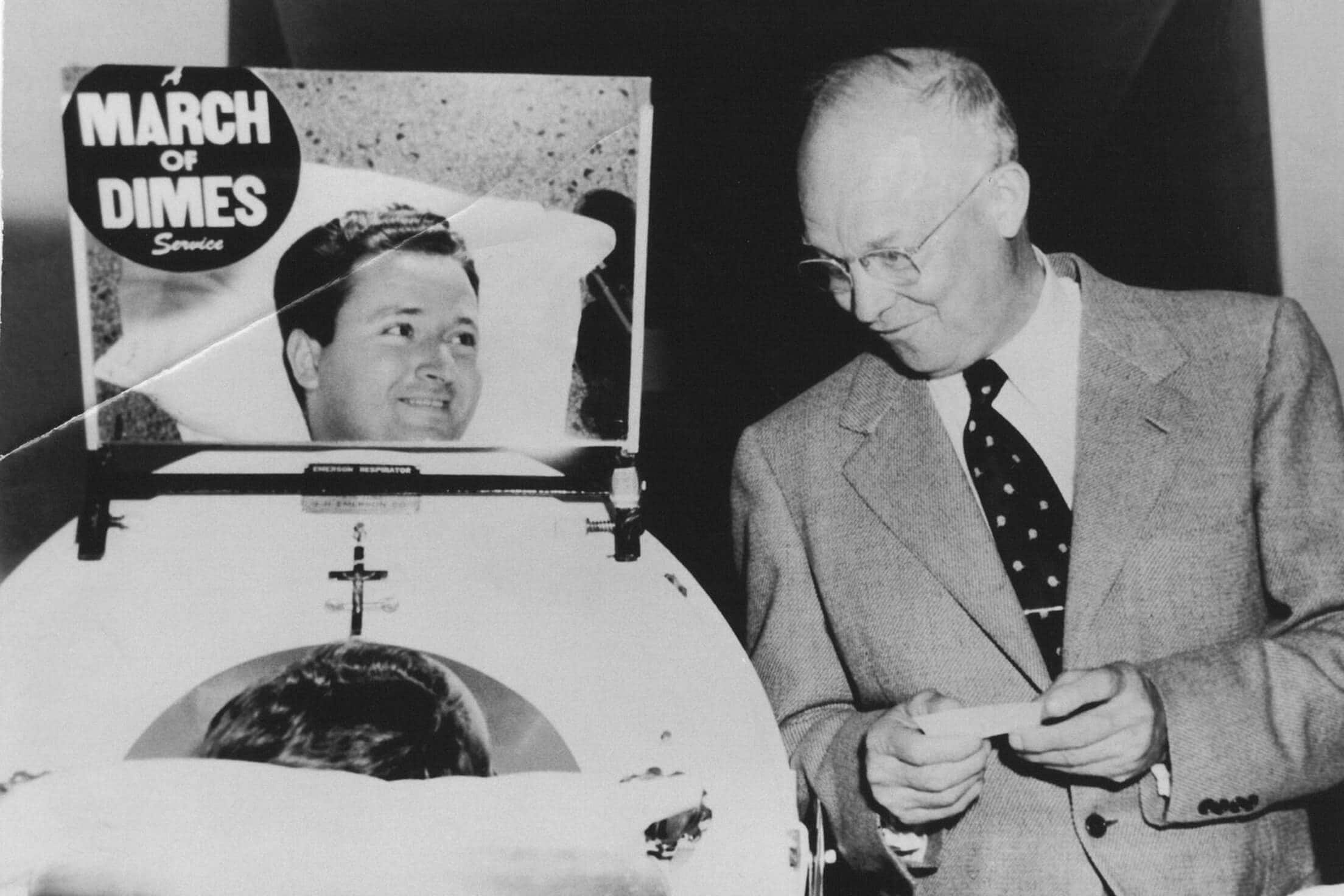In this black-and-white photograph, a scene from the 1950s or 60s unfolds, capturing a historical moment tied to medical history. On the right, an older man dressed in a gray suit adorned with a black tie featuring a white spot pattern stands attentively. He has rimless glasses perched on his nose and holds a small card with both hands. His gaze is directed downward, toward another individual. This second person is visible only through the reflection in a mirror attached to a large white pressure chamber, indicative of a tuberculosis treatment setting. The mirrored reflection shows a man who appears confined inside the chamber, with only his head and pillow visible. Above the patient, a sign reads "A March of Dimes Service," emphasizing the charitable involvement in combating this illness. The careful placement of elements and the creases in the photograph suggest it is a photo of a photo, adding a layer of authenticity and age to this compelling historical snapshot.